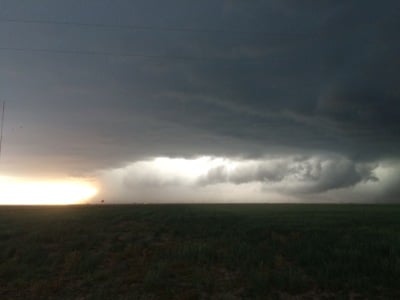The image captures a dramatic landscape scene dominated by an impending storm. The foreground features a vast, dark field with sporadic patches of green grass, hinting at a barren, almost desolate terrain. Above this field, the sky is cloaked in a thick, expansive blanket of ominous gray clouds, signaling the onset of severe weather, possibly a tornado or a hurricane. These clouds are darker, particularly on the right side, enhancing the stormy ambiance. In stark contrast, the middle section of the sky reveals a semblance of hope where light penetrates through the dense clouds, creating a break and illuminating the scene. This light has a warm, yellowish-orange glow, reminiscent of a sunset, adding a striking visual element to the otherwise gloomy setting. This powerful interplay of dark and light within the sky evokes a sense of awe and anticipation, making the image both dramatic and oddly comforting.